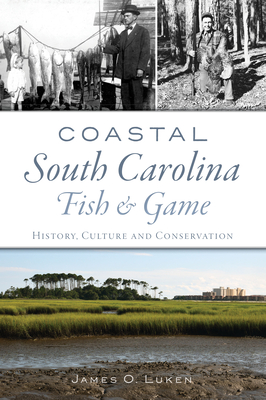The image depicts the front cover of a book titled "Coastal South Carolina: Fish and Game, History, Culture, and Conservation." The title, written in blue letters, is centered on a plain white background. Surrounding this title, the cover is divided into two sections with photographs: black-and-white images at the top and a large colored image at the bottom.

At the top left, a man dressed in a dark suit, black bow tie, white shirt, and dark hat stands beside a line of hanging fish. Beside him, a little girl in white watches the scene. To the right, another man smiles at the camera, seemingly holding a rifle, although the exact details are blurry. These top images are monochrome, adding a historical touch.

The bottom of the cover showcases a vivid colored image of a natural landscape. It features a muddy terrain leading to a small river or stream, bordered by medium-to-tall grasses and tall trees in the background. The sky is a blend of blue and white, and hints of buildings or potentially an industrial plant can be seen in the distance. The author's name, James O. Lucan, appears at the bottom, completing the detailed and evocative cover of the book.